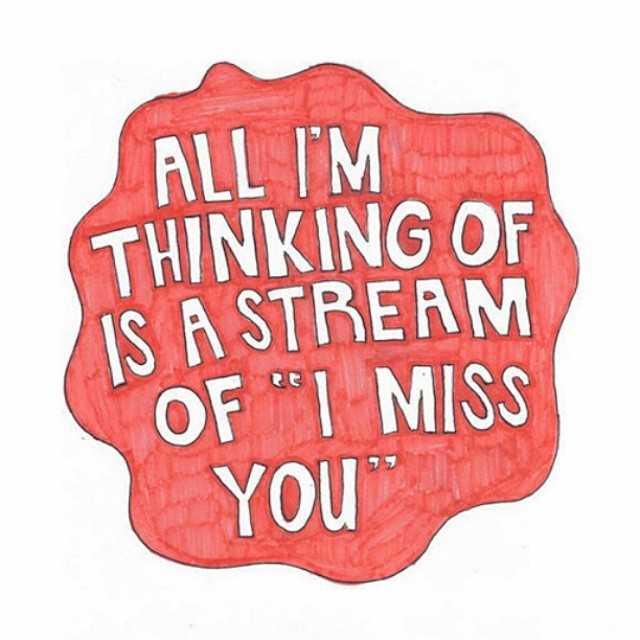The image is a hand-drawn text illustration featuring a wavy-edged circular shape resembling a splat or cloud. This shape is colored with a pink or rose hue, shaded vertically showcasing the texture of color pencil or crayon strokes. The central drawing is encased in a thin black outline, further emphasized by another black pencil outline tracing the outer perimeter of the pink wavy circle. Inside this shape, in all capital white block lettering, is the text: "All I'm thinking of is a stream of 'I miss you'," slightly uneven and slightly tilted, surrounded by a delicate black outline. The entire artwork rests against a pristine white background, giving it a floating appearance.